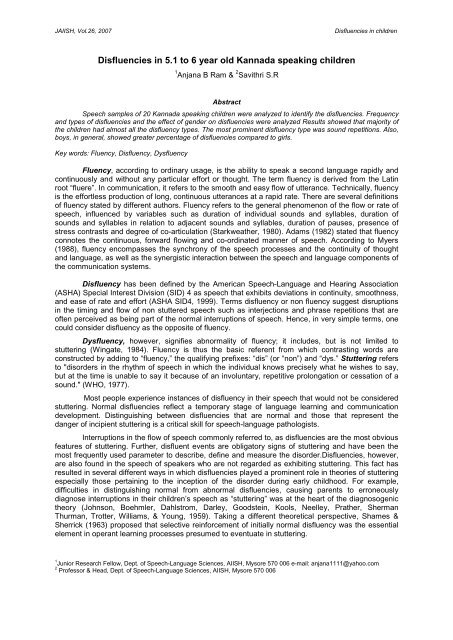The image displays a scan of an 11 by 14-inch sheet of paper, detailing a scientific study conducted on children. In the upper left corner, it notes "Javish, volume 26, 2007," indicating the source publication of the study. The upper right corner has the bolded title, "Disfluencies in Children," and below that, it specifies the focus of the study: "Disfluencies in 5.1 to 6-year-old Kannada-speaking children," with Kannada spelled as K-A-N-N-A-D-A. The page includes several paragraphs elaborating on the study's purpose, findings, and methodology, categorized under sections like "Abstract," which outlines the research scope and intent. The bottom of the page contains crediting notes and contact information for the researchers, possibly for further inquiries or correspondence. The document appears to be a critical academic paper, possibly a thesis, characterized by its detailed examination of fluency and disfluency in young Kannada-speaking children.